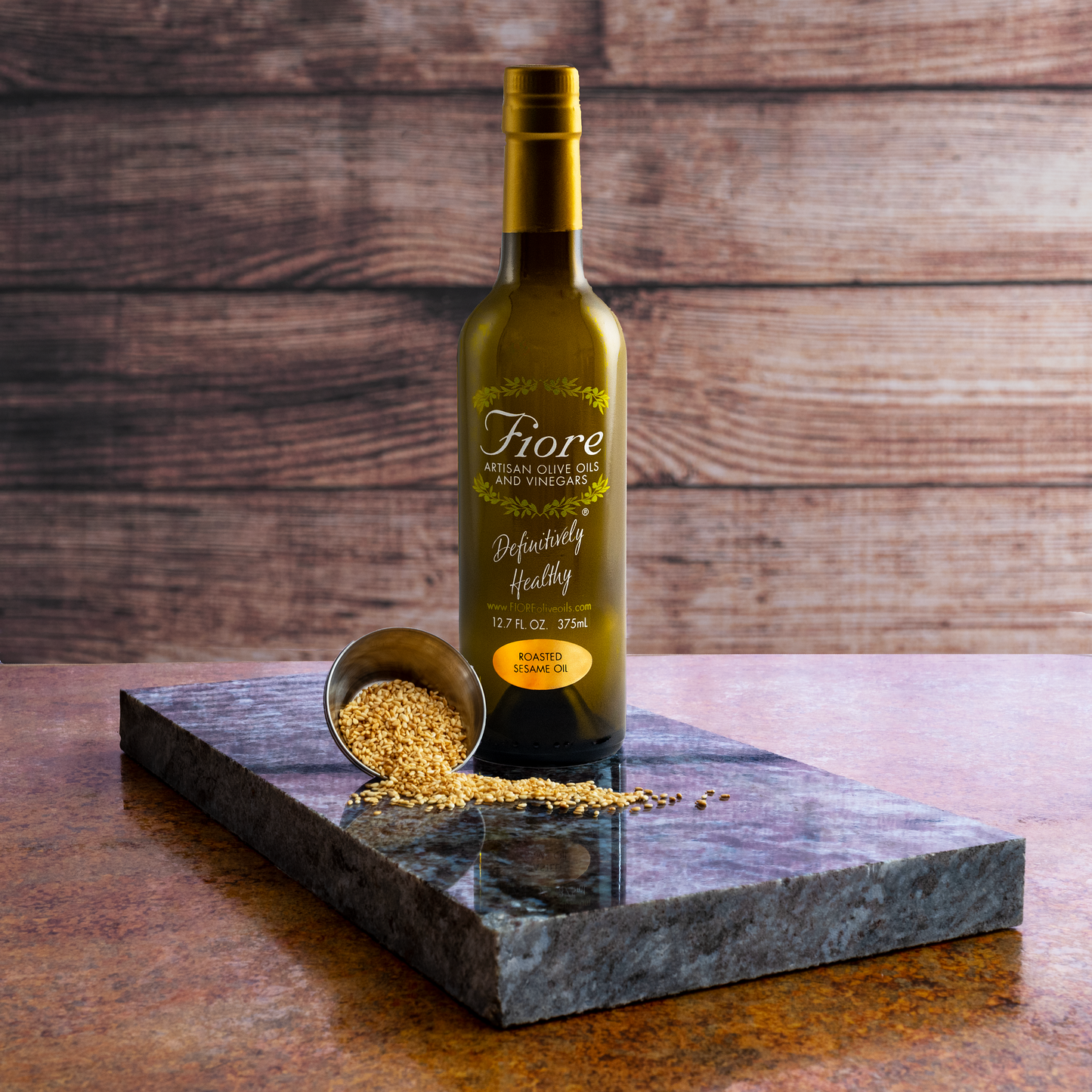This photograph prominently features a 12.7 fluid ounce bottle of roasted sesame oil from Fiore Artisan Olive Oils and Vinegars. The bottle is an elegant dark green hue with a dark gold foil wrapped around its top and lid, adding a touch of sophistication. The label on the bottle is detailed with white text that reads "Fiore Artisan Olive Oils and Vinegars," and it also proclaims "Definitely Healthy." This attractive bottle is centrally placed on a luxurious gray marbled rectangular slab.

The backdrop features a rustic brown wooden plank wall, enhancing the visual appeal of the presentation. The table surface beneath the marble slab is a brown countertop with subtle black veining, adding texture to the scene. Beside the bottle, a small, overturned silver bucket spills light brown sesame seeds onto the slab, adding an element of realism and inviting curiosity about the product. This image, with its professional composition and balanced elements, resembles an advertisement, showcasing the refined elegance and health-centric message of the Fiore brand.